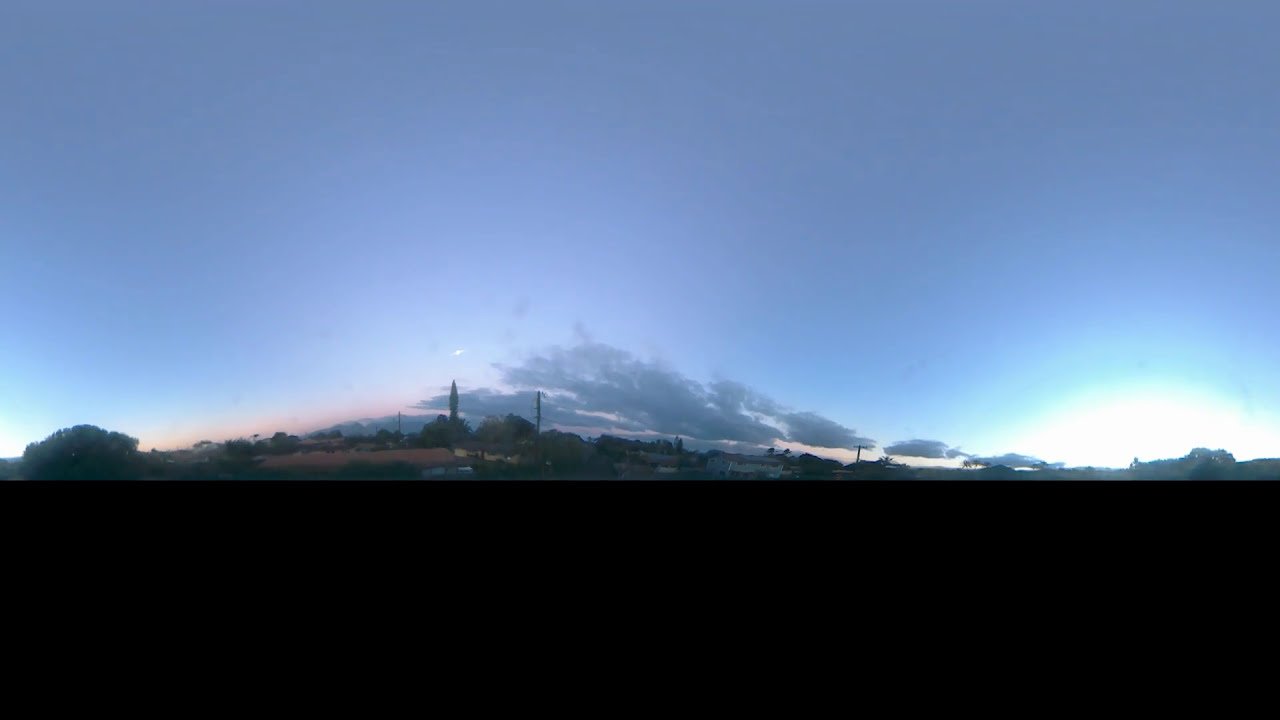The image captures a serene, expansive landscape at either sunset or sunrise, characterized by a vivid blue sky tinged with gray and purple hues, accentuated by wavy clouds drifting from right to left. To the right, a glowing sun is setting or rising, casting a beautiful white and orange glow in the sky. The ground, appearing almost pitch-black and flat, stretches out beneath the horizon, giving a surreal impression as if edited or viewed through a car window. In the distant backdrop, indistinct and hazy, lie possible monuments and signs of civilization, such as trees, power lines, and maybe even distant houses, adding to the mystique and depth of the scene. The overall effect is a stunning, albeit slightly warped, panorama that captures the tranquil beauty of the transitioning day.